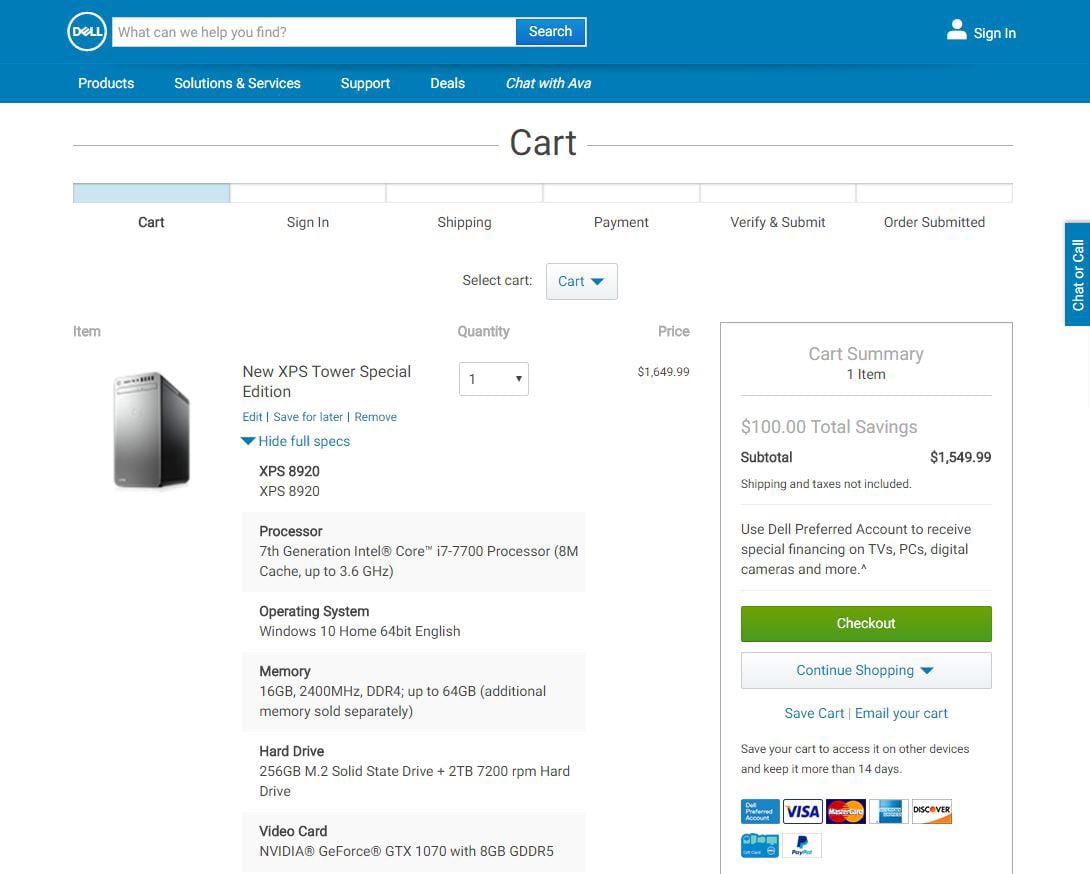The image shows a screenshot of the Dell website. At the top of the page is a blue banner, featuring a white search field with the text "What can we help you find?" and a blue search button. To the right of the search field is a white "Sign In" option next to a user icon. Directly beneath the banner is a navigation bar with white text, listing options such as "Products," "Solutions & Services," "Support," "Deals," and "Chat with AVA."

Below the navigation bar, the background turns white, featuring steps of the checkout process: Cart, Sign In, Shipping, Payments, Verify & Submit, Order Submit. Currently, the "Cart" tab is open. The cart contains one item: a new XPS Tower Special Edition. Options related to the cart item include "Edit," "Save for Later," "Remove," and "Hide Full Specs." The specifications section is expanded, displaying detailed information about the XPS 8920 model. Details include the processor, a 7th Generation Intel Core i7-7700 with 8M cache and up to 3.6 GHz speed, the operating system being Windows 10 Home 64-bit in English, and the memory specifications, which is 16 GB of 2400 MHz DDR4 RAM.